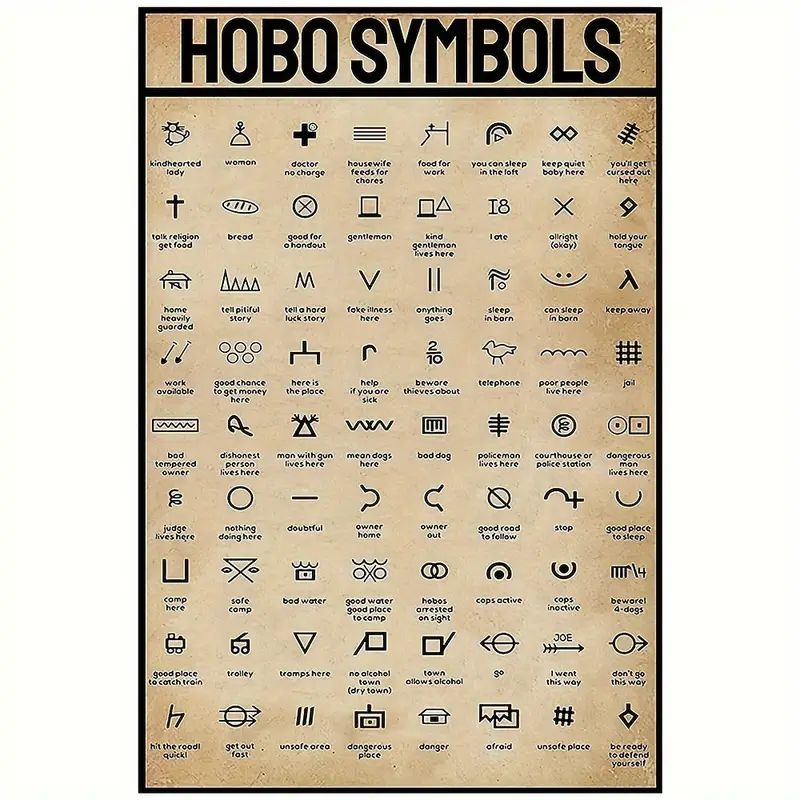This large, rectangular poster features a collection of Hobo symbols illustrated in black ink on a beige, aged background that may have once been white. The title "HOBO SYMBOLS" is prominently displayed at the top in black capital letters. The poster is meticulously organized into rows and columns, housing around 56 to 80 symbols, each accompanied by an explanatory caption. These symbols, used by hobos to communicate essential information, include various shapes like lines, birds, crosses, and squares. Each symbol conveys a unique message—such as a simple horizontal line meaning "doubtful," a bird representing "telephone," a cross indicating a place to receive food and religious aid, an X meaning "alright or okay," and a square denoting a "gentleman." The symbols offer insights into the hobo subculture, providing guidance on safe places, sources of food, active police presence, and more essential alerts.